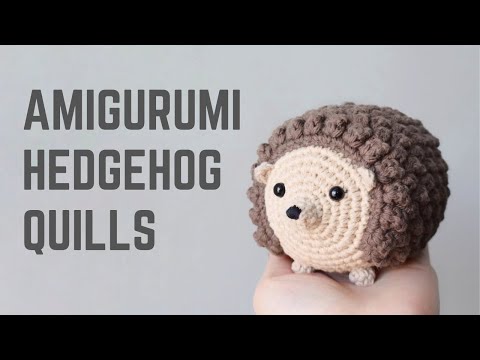The image has a landscape orientation with black letterbox bars occupying about 10-15% of both the top and bottom. The background features a medium gray color. On the left side, in dark gray, serif-less, all-capitals font, there are three lines of text reading "AMIGURUMI," "HEDGEHOG," and "QUILLS." Each word spans about 15% of the image's height. To the right, a hand emerges from the bottom, palm up and partially visible, holding a crocheted hedgehog in the Amigurumi style. The hedgehog faces the viewer with a smooth, pale, peachy face, two little ears, and two small feet. The main body is crafted with a brown bobble stitch, and it features two plastic eyes and a plastic nose.